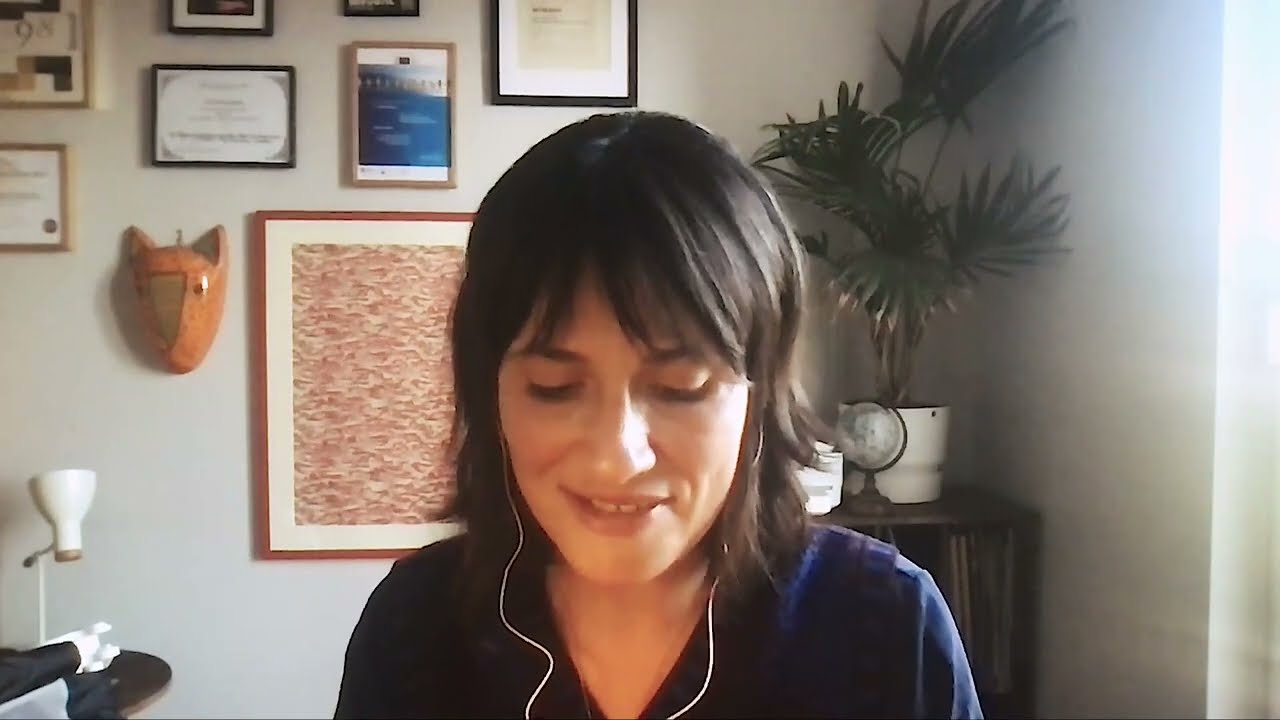This wide rectangular photograph features a young woman with short, dark brown hair that reaches just above her shoulders, styled with bangs. She is wearing white wired earbuds and a blue collared shirt. The woman is looking down, possibly smiling and appears to be speaking softly. Only the top half of her body is visible. In the background is the corner of a room, where the walls are painted a light gray-beige color. To the right side of the image, there is a brown coffee table with a tall green plant resembling a palm tree, housed in a white pot. The table also holds a globe. On the left side of the background, several framed pictures and documents hang on the wall, including what seems to be degrees and an abstract painting with red and light yellow colors. Additionally, there is a metal fox head wall decoration and the partial view of a lamp and possibly a seat. The overall setting is well-lit, indicating sunlight streaming into the room.